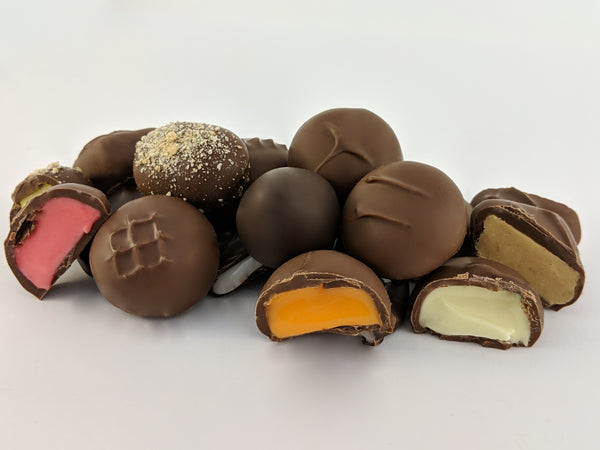This photograph showcases a small pile of assorted bonbons against a white background. The arrangement primarily features milk chocolate-covered bonbons, with a few notable exceptions that add diversity to the collection. In the foreground, three bonbons have been cut or bitten to reveal colorful fillings: a bright pink one, a vivid orange one, and a creamy white one that appears goopy. Another bonbon with a tan peanut butter filling is also cut, while one in the pile is dusted with chopped nuts or toffee bits. Positioned centrally is a dark chocolate bonbon, surrounded by various roundish milk chocolate pieces, some adorned with intricate chocolate designs including a square-like pattern. Notably, there is a milk chocolate bonbon with a bite taken out that reveals a bright pink, non-liquid filling. The arrangement, overall, displays a rich variety of textures and flavors, with the chocolates neatly laid out, giving a detailed glimpse into their tempting insides.